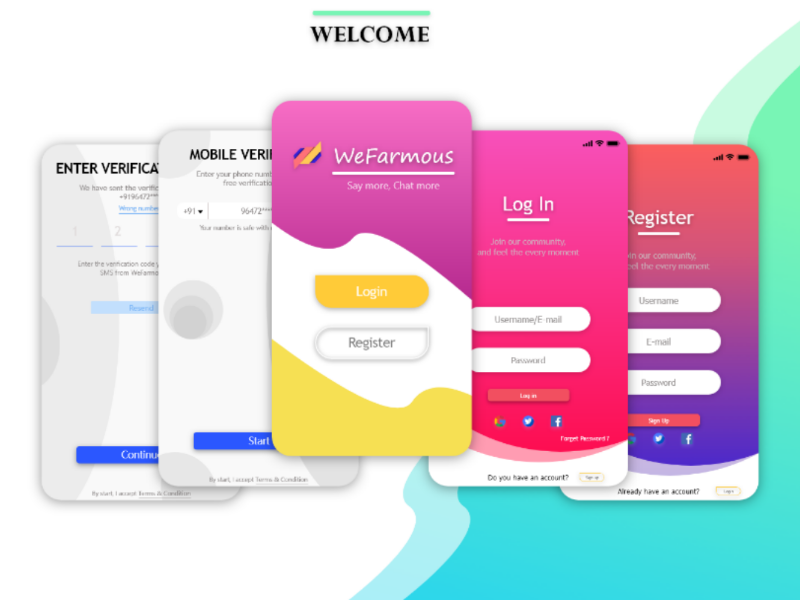The image is a vibrant and engaging welcome graphic centered around mobile interface designs. At the top, a prominent blue bar runs across the center, leading directly to the word "Welcome" elegantly rendered in black text beneath it. Central to the image are five distinct mobile screen mockups, artfully stacked and slightly overlapping each other.

Starting from the left, the first screen features a white background with text indicating "Enter Verification," although partially obscured by the subsequent screen. The next mockup prominently displays the word "Mobile," but the remainder of the text is cut off. This too has a white interface.

Occupying the center position, the third screen showcases an app titled "We Farm Us," with the catchy phrases "Say More, Chat More" displayed over a dynamic purple, white, and yellow design. Moving right, the fourth screen presents a lively red-to-pink gradient backdrop, featuring input fields for "Username," "Email," and "Password," alongside a "Login" button, all in white text.

The fifth and final screen on the right exudes a bold gradient transitioning from purple and blue to red, with "Register" at the top and three input fields for "Username," "Email," and "Password," accompanied by a "Sign In" option.

Additionally, a green-to-blue patterned design fills the bottom corner on the right side of the image, adding a splash of color and balance to the overall composition.